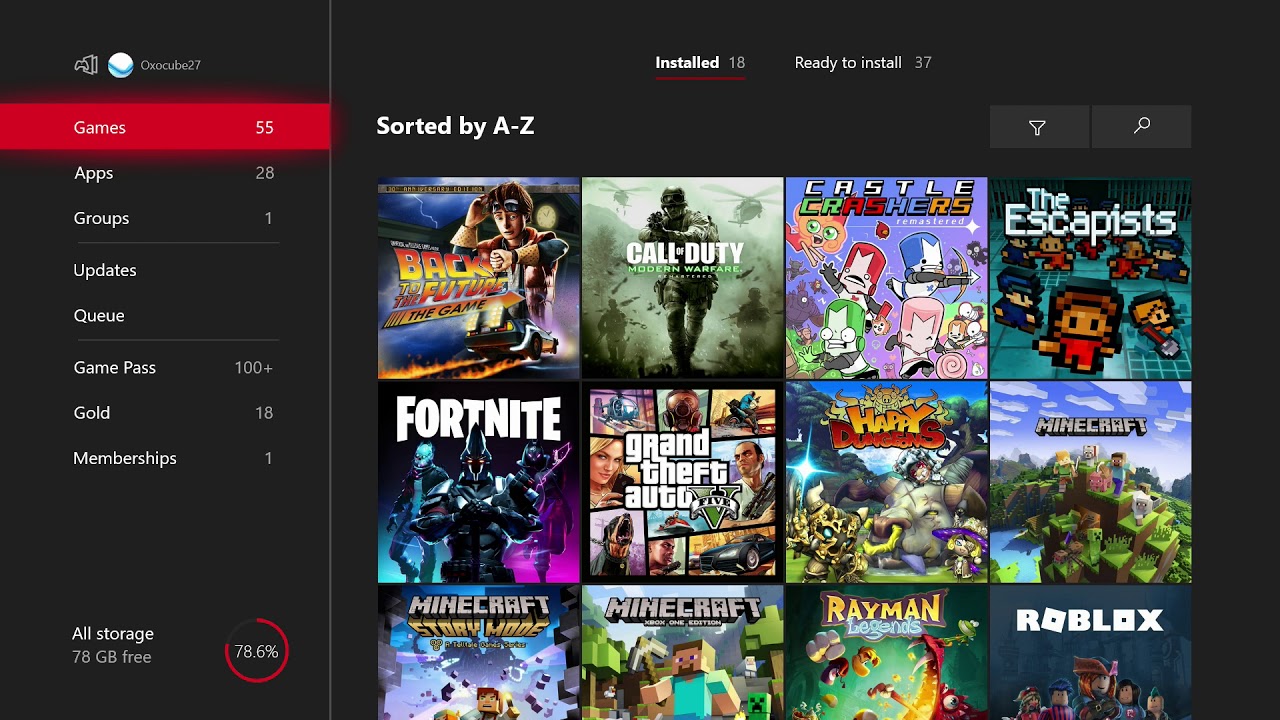This is a detailed cropped screenshot of a gaming console's home page set against a black background. In the top left corner is a small, black-and-white icon resembling a PlayStation. Adjacent to the icon is a profile picture, accompanied by the account name in very small white letters to its right. Below this, on the left side, is a vertical navigation menu listing categories such as Games, Apps, Groups, Updates, Queue, Game Pass, Gold, and Memberships. At the bottom of this menu, it says "Add Storage" or "All Storage," followed by a note indicating 76 GB of free storage.

The bottom right corner features a circle, nearly filled in red, with the text "78.6%" in its center, displaying storage usage. At the top center of the page, "Installed 18, Ready to Install 37" is written in small white letters, providing a summary of the game installations and pending installations. Towards the top left corner, "Sorted by A to Z" is displayed, organizing the content in alphabetical order. The main section shows a grid of square thumbnails featuring video game covers, arranged in four rows with four covers per row, giving a clear view of the available games.